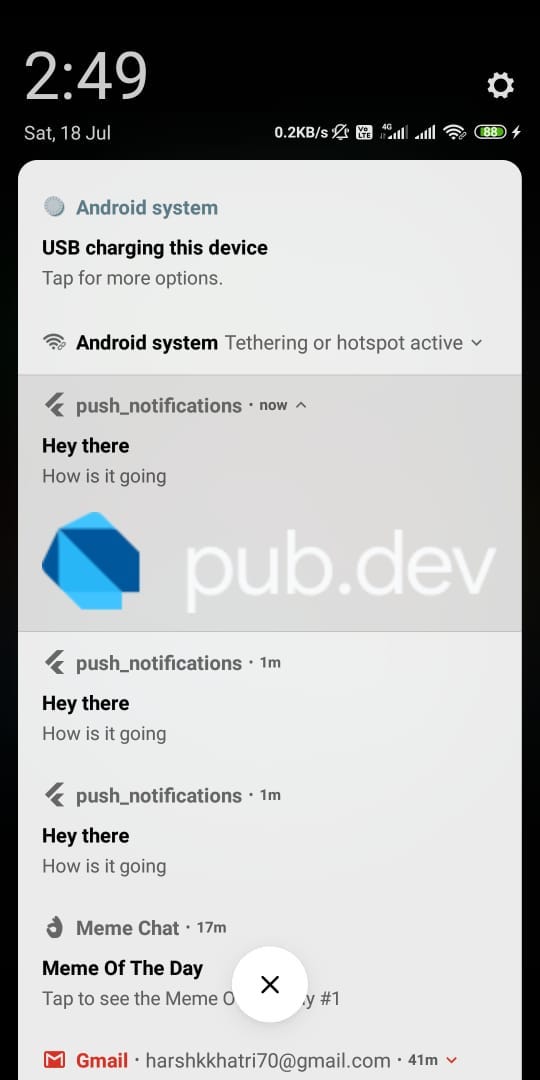The image is a screenshot taken from a cell phone displaying the notification and status bar. At the very top left corner, it shows the time "2:49" on a Saturday, dated "18 JUL." To the right, there is a settings wheel icon followed by "0.2 KB/s" and a series of status icons indicating LTE, 4G connectivity, full signal bars, a Wi-Fi signal, and an 88% battery life with a lightning bolt, all set against a black background.

Within this black background is a large white-gray rectangular section containing multiple notifications in separate rows. The first row features a bullet point labeled "Android system" in light blue, followed by "USB charging this device" in bold text. The next row contains the instruction "tap for more options." A subsequent row includes a Wi-Fi signal icon and the text "Android system tethering or hotspot active" with a drop-down arrow.

Another section is highlighted in gray, stating "Push notifications now" with an upward arrow. Following this, another message reads "Hey there," in bold, followed by "how’s it going?" Each line appears in separate rows.

Further down, there is a symbol in a combination of light and dark blue followed by "pub.dev" in large white text. Another series of notifications follow, each in separate rows: "Push notifications 1M" with the repeated phrase "hey there, how’s it going?" in bold.

An "okay" hand symbol is shown, followed by "meme chat 17M" and a new row with the bold text "meme of the day," followed by "tap to see meme of," which is partially obscured by a white circle with an X.

At the bottom, in red, there is the Gmail logo followed by "Gmail," an email address "h-a-r-s-h-k-k-h-a-t-r-i-70 at gmail.com," and "41M" with a down arrow to indicate more options.